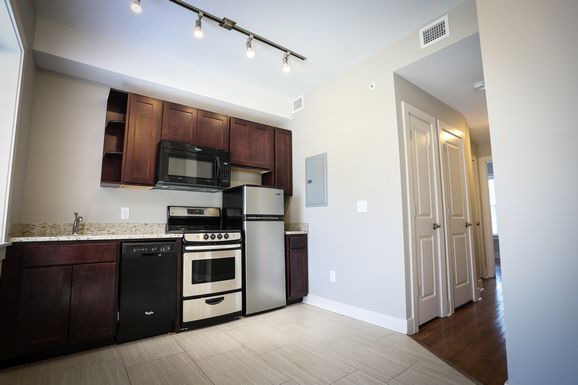The image appears to capture a well-lit, modern apartment kitchen and part of the adjoining hallway. Taken from a camera, the photo showcases an open-concept kitchen layout without any black accents. Visible in the hallway are two narrow white doors, likely closets, positioned close together and surmounted by a vent. Another vent is visible on the same wall, above an electric panel located near the gray-colored cabinets.

The baseboards along the walls are painted white, providing a crisp contrast to the wooden stain of the kitchen cabinets. A microwave is integrated above the stove within one of the cabinetry sections. Adjacent to this is a countertop extending to a space beneath it that houses a dishwasher. The cabinets feature doors, adding to the ample storage space available in the kitchen.

The flooring in the kitchen itself is gray with a panel design, distinct from the wood-colored flooring seen in the hallway area. Light streams in from a window situated at the corner of the hallway, indicating it is daytime. The kitchen ceiling features four recessed lights, ensuring the area is brightly illuminated. Overall, the scene depicts a tidy and contemporary living space.